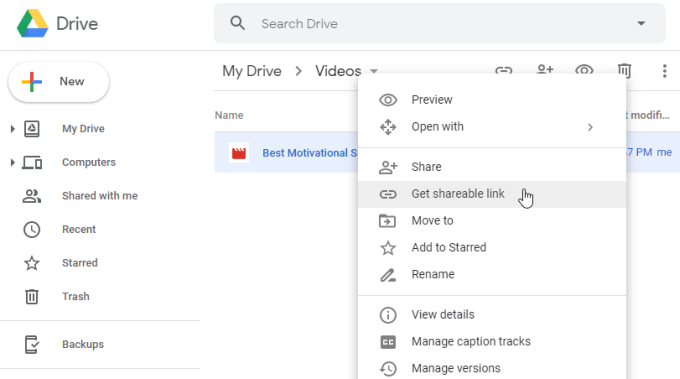A screenshot displaying the Google Drive interface. In the upper right corner, the Google Drive logo is prominently displayed with the word "Drive" next to it. Spanning across the top, there is a search bar featuring a magnifying glass icon and the text "Search Drive." 

On the left side, a vertical column lists various options: 
1. A highlighted "New" icon marked by a plus sign.
2. Below it, "My Drive" accompanied by an icon.
3. An icon of a computer labeled "Computers."
4. An icon depicting two people with the text "Shared with Me."
5. An icon of a clock with the label "Recent."
6. A star icon next to "Starred."
7. A trash can icon alongside "Trash."
8. At the bottom, a rectangle with a checkmark identified as "Backups."

Superimposed on the main interface, a smaller window shows additional options:
1. An eye icon labeled "Preview."
2. Four arrows pointing in different directions with the caption "Open With."
3. A person and plus sign icon labeled "Share."
4. An icon resembling a paper clip with the text "Get Shareable Link."
5. A folder with an arrow labeled "Move To."
6. A star icon labeled "Add to Starred."
7. A pencil icon alongside the label "Rename."
8. A circle with an eye icon and the text "View Details."
9. A square with the letters "CC" and the caption "Manage Caption Tracks."
10. A circular arrow icon labeled "Manage Versions."